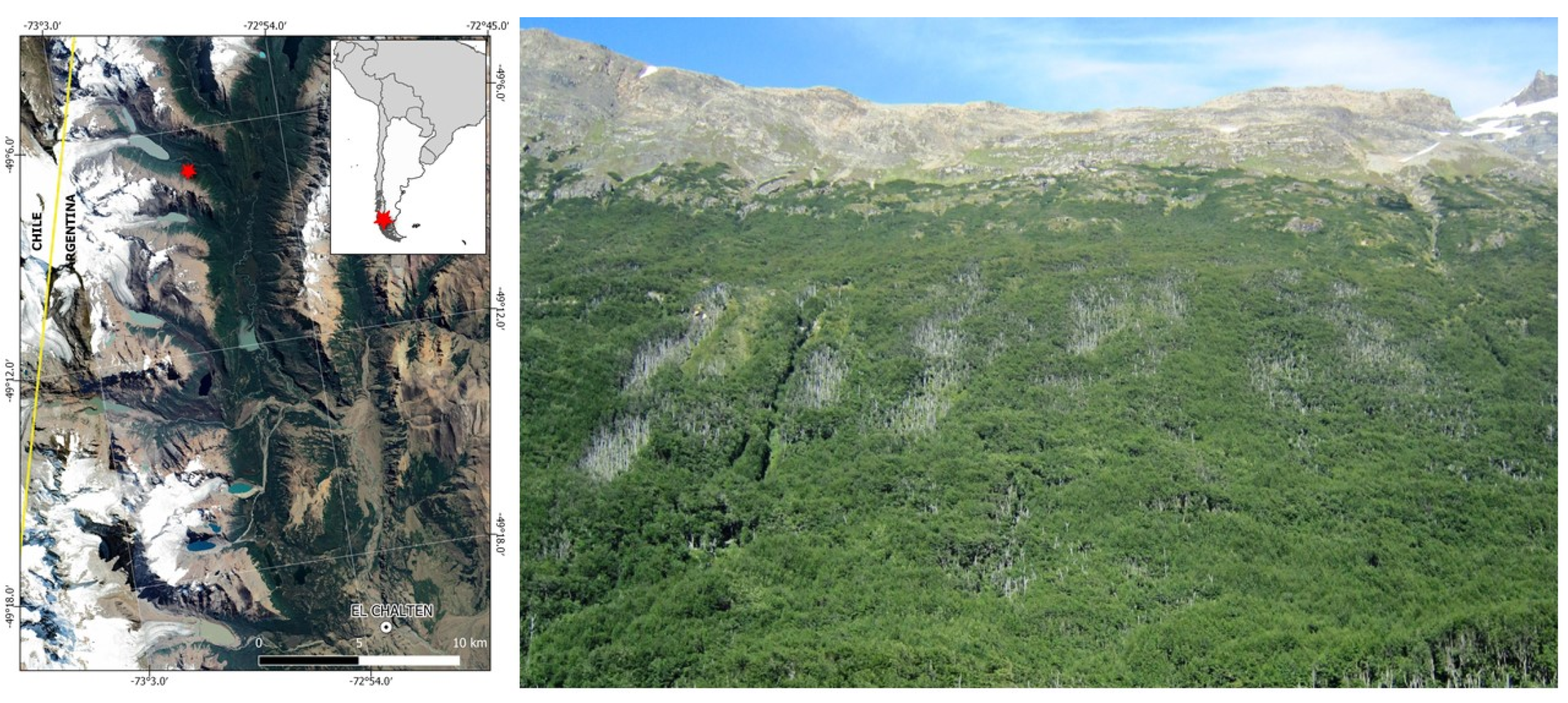This composite image pairs a detailed topographic map with a vivid photograph of a picturesque mountainous region. The left one-third of the image displays a satellite view of a snow-capped mountain range interspersed with large green sections: likely forests or vegetation. A prominent red dot marks a location adjacent to a large blue body of water. Overlaid on this detailed map is a smaller inset map showing the broader context, locating this specific geographic area in the southern part of South America. 

The topographic map exhibits various altitudes and terrains in a hand-drawn or digitally-rendered style. In the upper right corner of this section, a smaller map provides an overview, pinpointing where this detailed snapshot fits within the continent.

The right two-thirds feature a stunning photograph of the described mountainous terrain. A steep cliff extends upwards from a lower elevation in the front to a higher peak in the background. The mountain is blanketed with lush green trees and dense vegetation, except for scattered patches of barren ground that lack greenery, potentially indicating rocky outcrops or dead patches. The top of the cliff shows a mix of snow and rocky formations, with the left side covered more sparsely compared to the right. Above, a clear blue sky forms a striking backdrop to the rugged beauty below, emphasizing the wild and untamed nature of this expansive, scenic area.